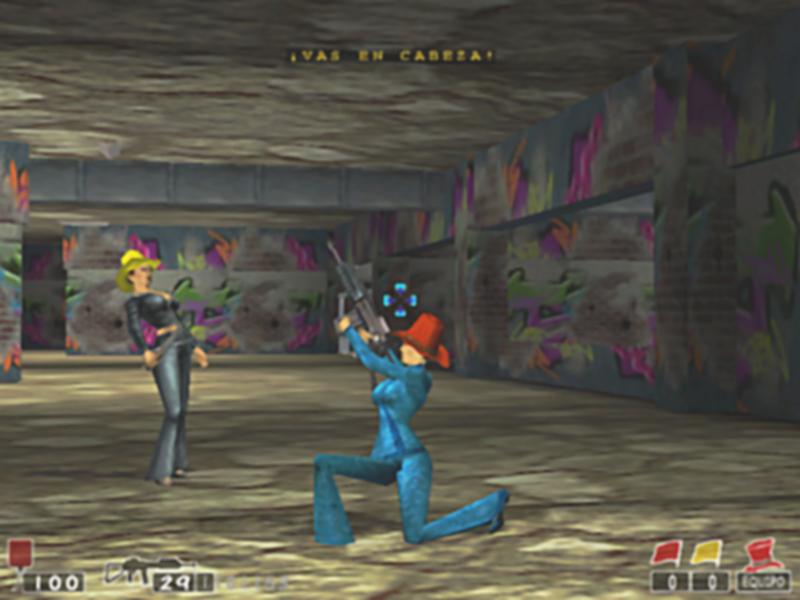Screenshot from a late 90s or early 2000s video game, characterized by its blocky and non-realistic graphics. In the bottom left-hand corner, two icons are present— a red square with the number "100" beside it, and a small gun with "29" next to it. The bottom right-hand corner displays three other icons— a red flag with the number "0" beneath it, a yellow flag, and a red top hat with the word "round" underneath. Text in Spanish appears in the upper center of the screen. The game environment includes a grainy, low-resolution stone floor and graffiti-like walls. Two female characters are visible: one on the left wearing a yellow hat and a black pleather outfit, and another in the front holding a giant gun, adorned in a red cowboy hat and a blue one-piece outfit.